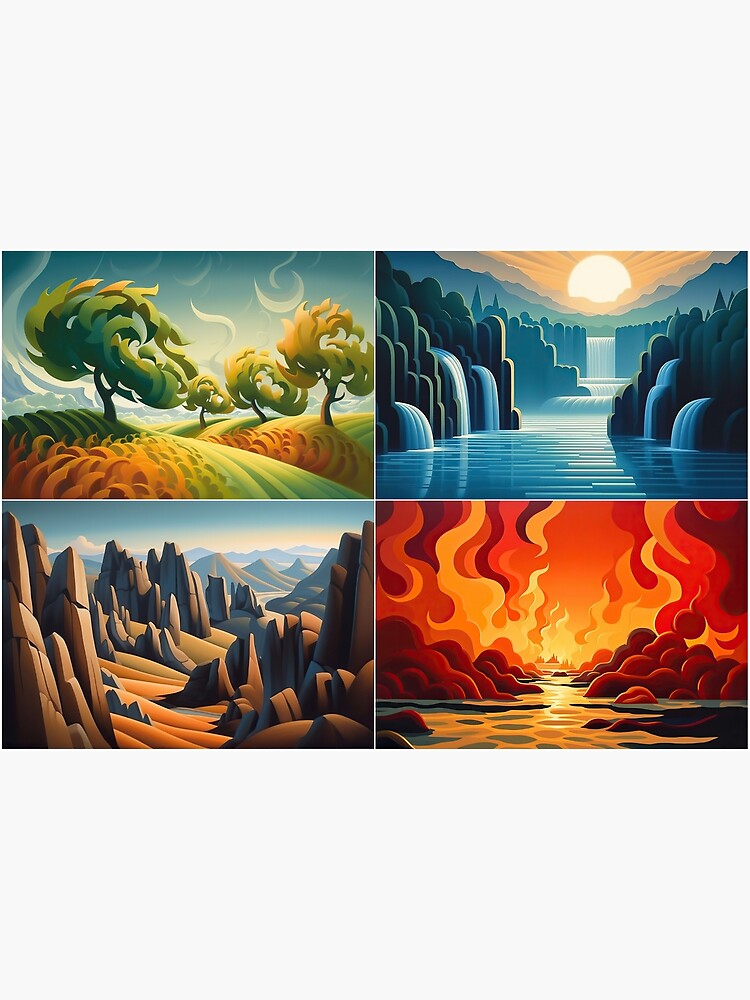This image consists of four distinct, rectangular illustrations arranged in a 2x2 grid, each vividly depicting one of the natural elements in a stylized, possibly computer-generated, cartoonish vector style.

**Top Left:** This illustration represents **wind**. It depicts four stylized trees swaying dramatically on rolling green hills interspersed with orange grasses. The background includes white swirls in the sky, symbolizing powerful gusts of wind. Each tree varies in size and placement, indicating depth and movement.

**Top Right:** The central focus here is **water**. This image presents a serene lake or river with a large waterfall at the distant center. Surrounding the waterway, several smaller waterfalls cascade down dark, rounded stone hills on both sides. The scene is bathed in blue tones, with a setting sun casting a peachy glow over the horizon, blending into an orange and blue sky.

**Bottom Left:** Illustrating **earth**, this picture showcases a barren, rocky landscape akin to a desert or the Grand Canyon. Jagged, tall brown rocks dominate the scene, with an orange dirt path running through them. Distant mountains are visible under a clear blue sky, highlighting the vastness and aridity of the terrain.

**Bottom Right:** This fiery depiction of **fire** suggests volcanic activity. Dominated by intense flames of red, yellow, orange, and maroon, the image features a lava pool at its center. Surrounding the flames are dark, rounded rocks, with water visible in the foreground, creating a stark contrast between fire and the other elements.

Together, these four illustrations form a cohesive representation of the elements—wind, water, earth, and fire—each strikingly distinct yet harmoniously integrated into a single, detailed, evocative image.